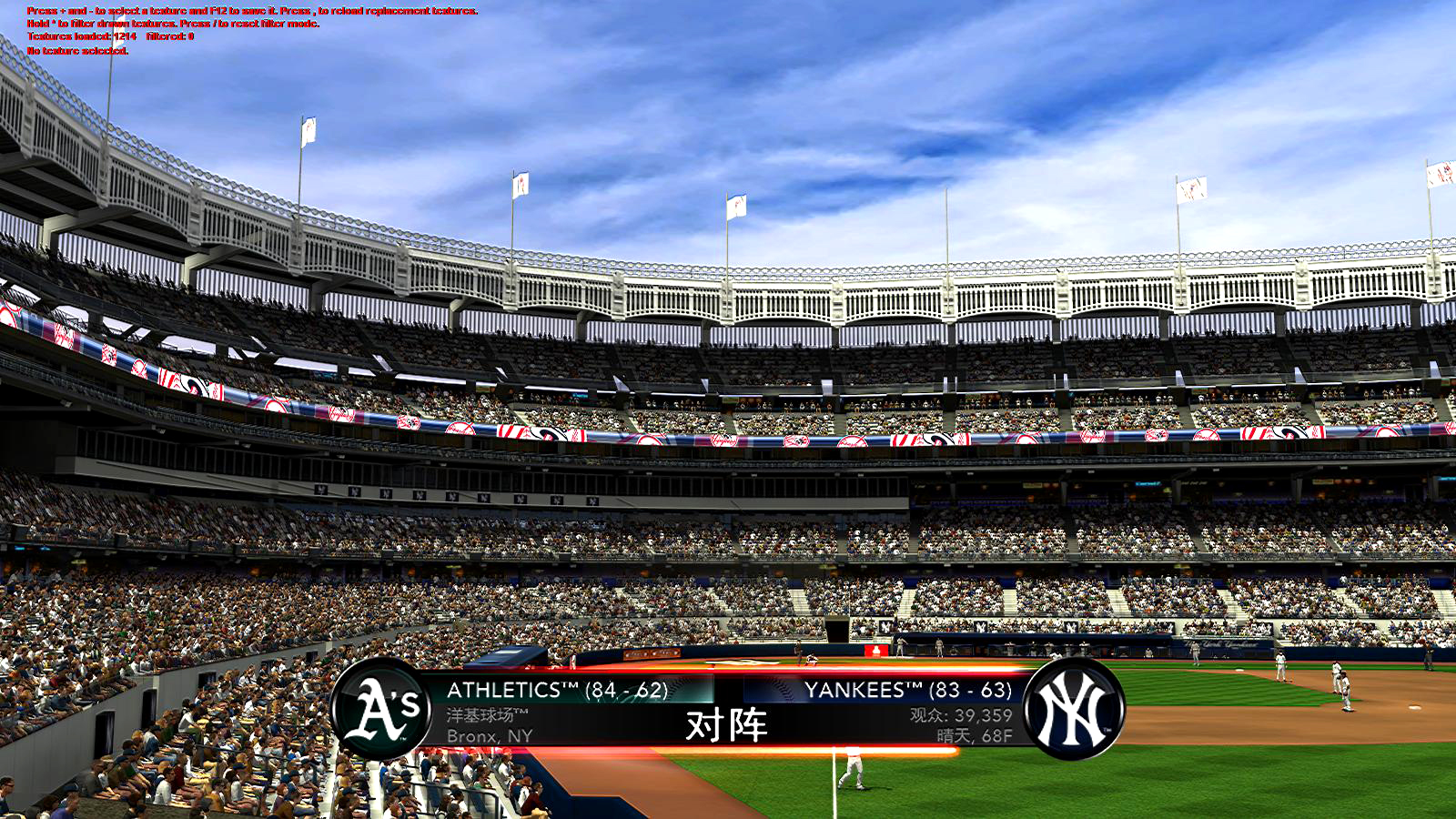The image depicts a bustling stadium filled with enthusiastic fans, layered with five distinct levels of seating. This stadium is presumably Yankee Stadium, identifiable by the competing teams on the field: the Athletics, represented by an "A's" symbol in a circular design and boasting a seasonal record of 84-62, and the Yankees, denoted by their iconic interlocking "NY" logo and a record of 83-63. The central grassy area of the baseball field is vibrant and meticulously maintained, with several players visibly positioned near the bases. The sky overhead is a striking blue, adorned with delicate, wispy clouds. At the topmost edge of the stadium, a series of approximately seven white flags can be seen fluttering in the breeze. Additionally, some red printed computer coding is faintly visible in the top left corner of the image, adding a curious element to the scene.